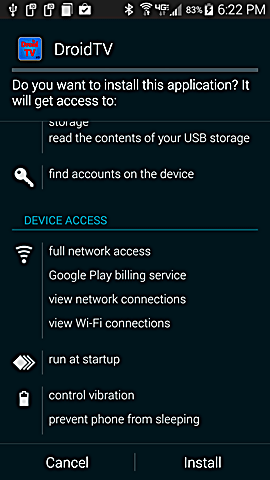This image is a detailed screenshot of a mobile device's application installation prompt. The top of the image features a black status bar displaying several icons: a white pitchfork-like symbol, two phone icons with square outlines, two layered squares, a shopping bag with a check mark, Bluetooth symbol, Wi-Fi symbol, 4G signal strength indicator, showing strong connectivity, a battery indicator at 83% charge, and the time displayed as 6:22 p.m.

Below the status bar, a red and blue icon is visible with the text "Droid TV" next to it in white font against a blackish-blue background. Proceeding downward, there's a gray bar followed by a prompt that reads, "Do you want to install this application?" It mentions that the app will gain access to storage and details specific permissions, such as reading the contents of USB storage.

Subsequently, a key icon is displayed next to the text, "Find accounts on the device." Further down, in blue font, the title "Device Access" is shown alongside a blue line. Below this, there is a list of permissions including: "Full network access," "Google Play billing service," "View network connections," and "View Wi-Fi connections," each accompanied by respective icons—a Wi-Fi symbol resembling a funnel with a dot at the bottom.

The permissions continue with "Run at startup" illustrated by blue layered boxes, "Control vibration," and "Prevent phone from sleeping," complemented by a battery icon. A thin gray line runs across the screen, dividing the permissions area from the action buttons.

At the bottom of the screenshot, there are two options: "Cancel" and "Install," displayed in white font and separated by another thin gray line. The overall visual quality of the image is clear with no other significant objects present.